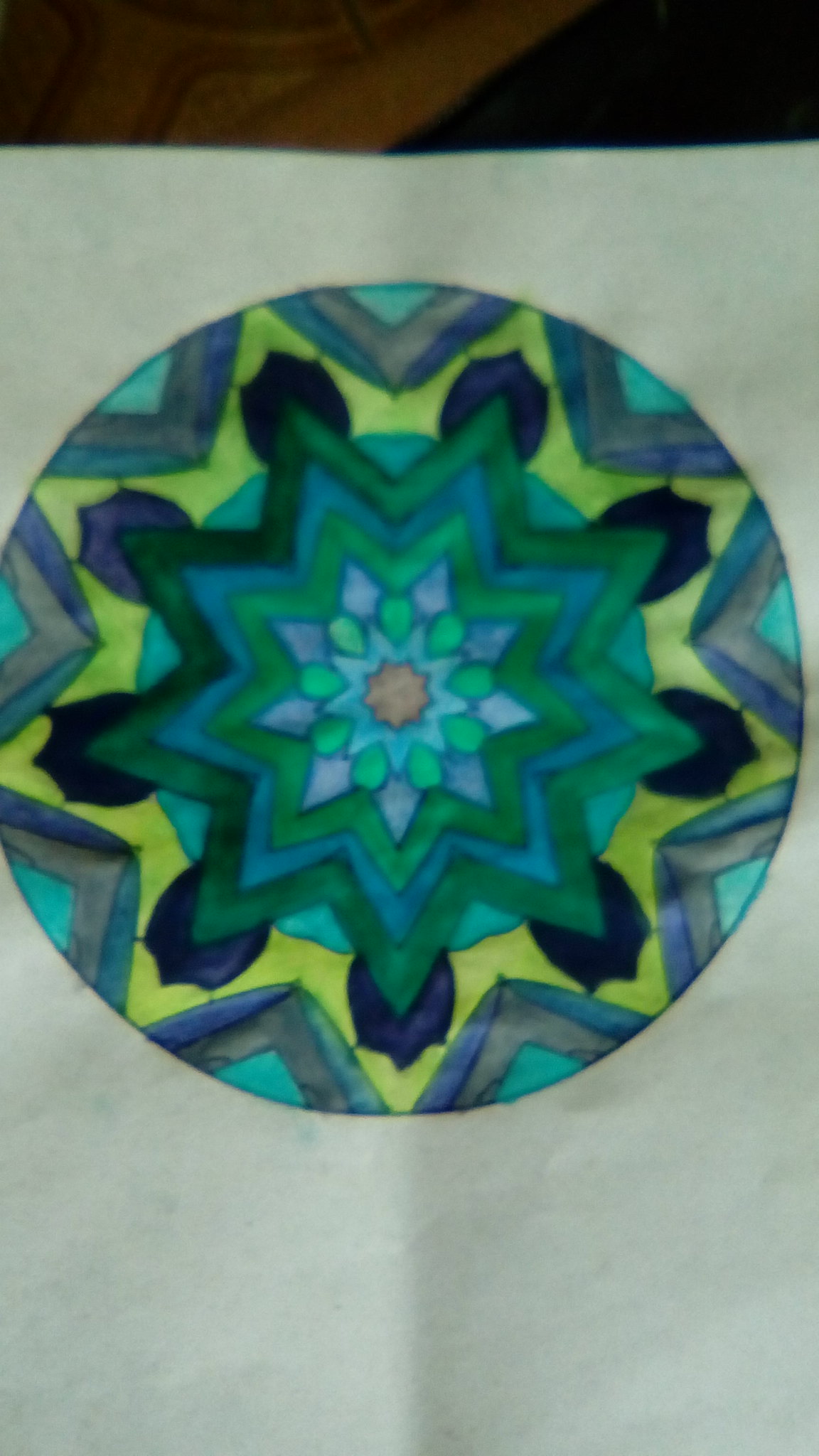The image features a detailed artwork rendered on what seems to be thin, off-white sketch or crafting paper. Dominating the piece is a large, circular form defined by a series of concentric, zigzagging lines. These lines create a star-like pattern that emanates from the center. The outermost lines are adorned with vibrant hues of blue and purple, which transition into shades of yellow and green as they move inward. Various smaller shapes, colored in green and orange, populate the center of the composition, contributing to its intricate design. The artwork stands alone with no accompanying text.